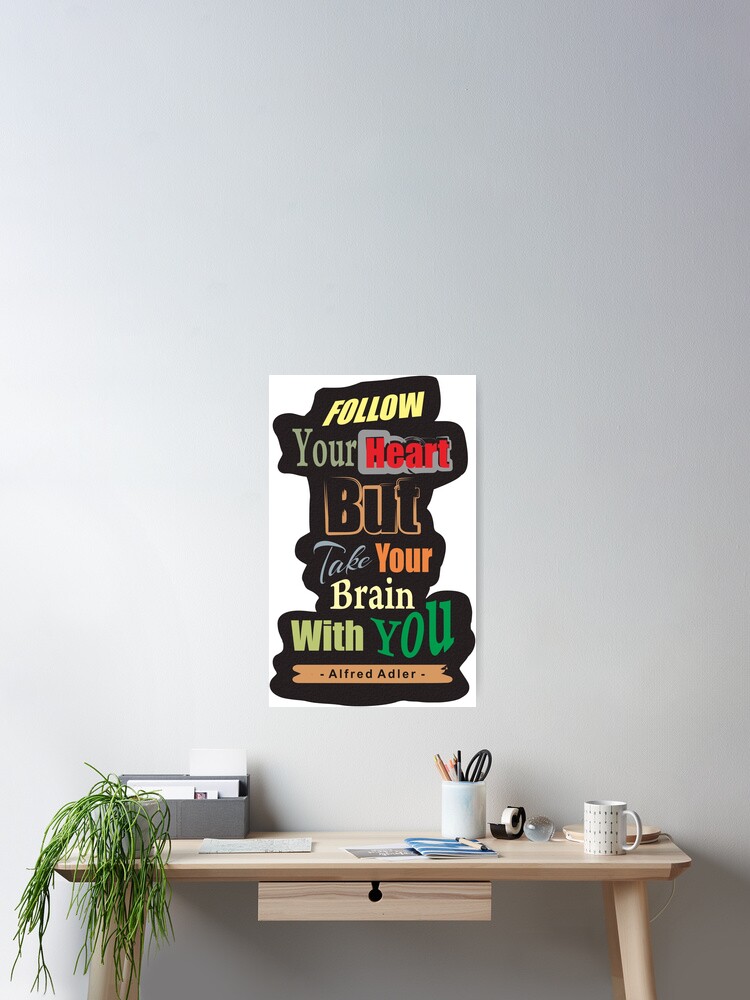The image depicts a vertically aligned, indoor setting featuring a small, thin desk made of light-colored wood or laminate, positioned against a white wall. The desk, possibly handmade, has a single drawer beneath it and stands on four legs, though only two are visible due to the angle. 

Above the desk, a white poster with a black outline displays the multicolored text: "Follow your heart, but take your brain with you" — attributed to Alfred Adler in black text at the bottom. 

On the desk, a neatly arranged array of items includes a white desk lamp with a long arm, a white coffee cup with a pattern, a pencil holder filled with pencils and scissors, a tape dispenser, and several thin brochures or books. To the left, a potted plant with thin, drooping green leaves sits beside a gray box that likely contains letters or envelopes.